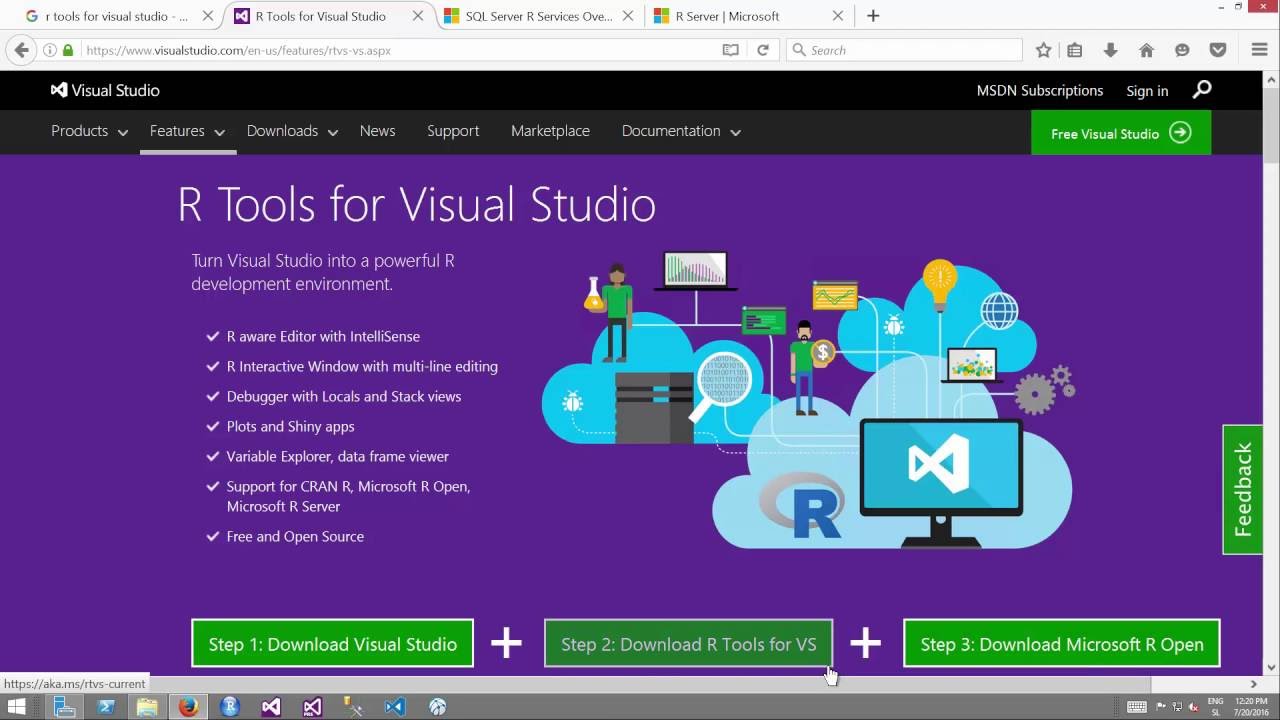The screenshot depicts a browser page with four tabs visible at the top. The tabs are listed as follows: 

1. Tools for Visual Studio
2. Tools for Visual Studio (selected)
3. SQL Server Services
4. Server Microsoft

The displayed browser page, whose specific browser is unidentified, focuses on "Tools for Visual Studio." 

At the top of the page, there's a black horizontal navigation bar featuring options such as Visual Studio, MSDN subscriptions, Sign In, and a search icon. Below this, a secondary navigation menu includes seven tabs: Products, Features, Downloads, News, Support, Marketplace, and Documentation. To the right of these tabs, a green button labeled "Free Visual Studio" is prominently displayed.

The main content area occupies the majority of the screen, characterized by a purple background. It highlights "R Tools for Visual Studio," showcasing a large list with check marks indicating various features. These tools are designed to transform Visual Studio into a robust development environment for R, a programming language primarily used for statistical computing. Some listed features include an R-aware editor with IntelliSense and an R interactive window.

On the right side of this purple section is an engaging graphical illustration depicting people utilizing these tools, featuring screens, gears, and other elements symbolizing the development process.

At the bottom of the purple area, there are three green boxes with instructions to get started:
1. Download Visual Studio
2. Download R Tools for Visual Studio
3. Download Microsoft R Open